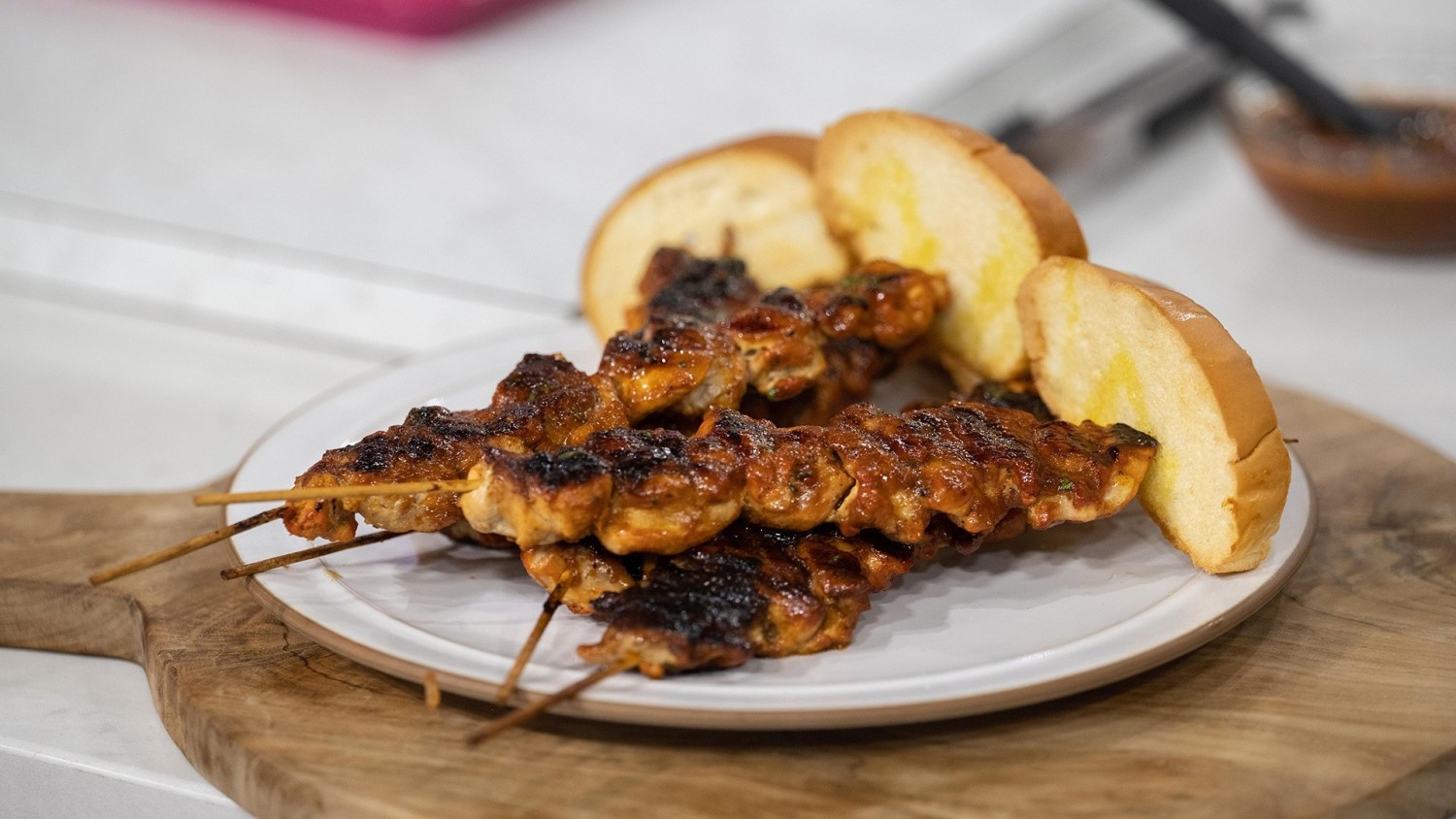On a round white plate with a brown rim, approximately five to six grilled meat shish kebabs lie stacked upon each other. Each kebab is skewered with a visible brown stick and exhibits caramelized tones with some charring, indicating they could be lamb or chicken. Accompanying the shish kebabs on the plate are three slices of toasted bread, either French or wheat, arranged to stand on their side resembling a small wall and likely drizzled with butter or honey. The plate is placed on a round wooden paddle serving board with a long handle, all situated on a white countertop. In the background, there is a blurry white bowl with a ladle and a brownish liquid, possibly barbecue sauce.